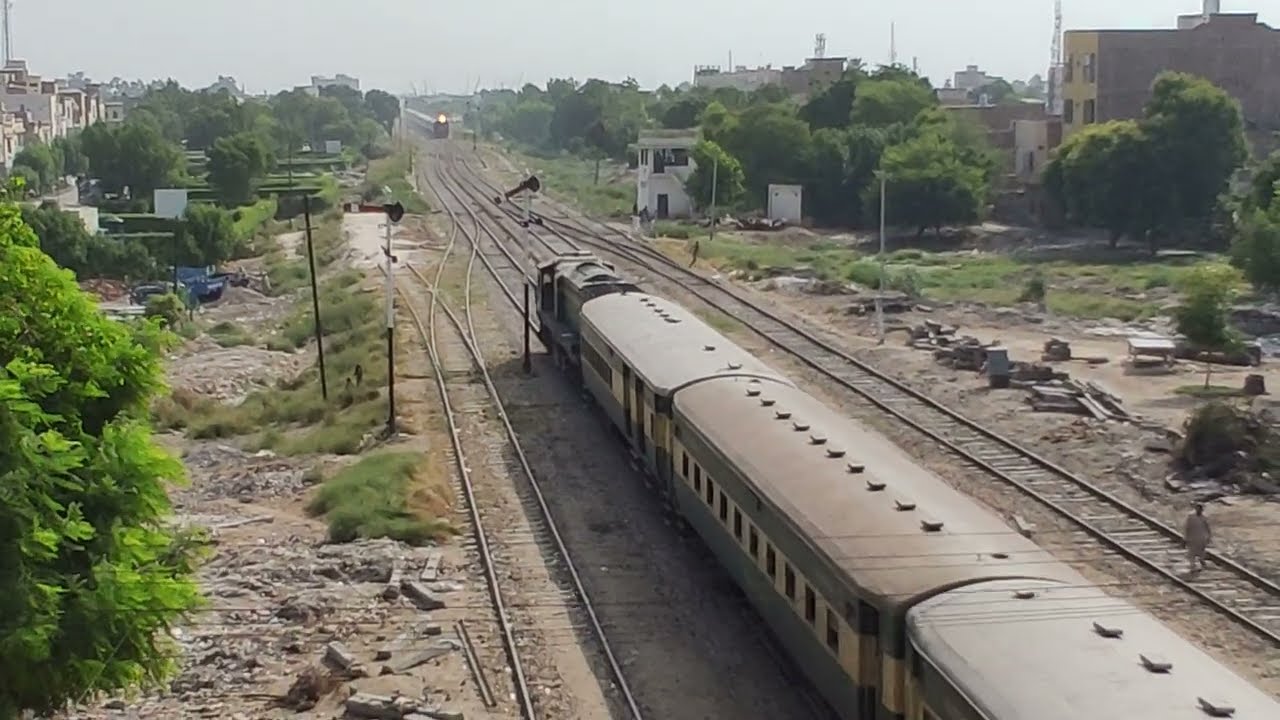The photo provides a detailed overhead view of a train yard on a clear day. In the foreground, a passenger train with three cars, possibly a locomotive or caboose, is moving away from the camera along one of the three visible tracks. Adjacent to these tracks, on the right, a person dressed in light-colored clothes is dangerously walking down the middle of an empty track. In the distance, another train is approaching, identifiable by its single headlight. The area is cluttered with assorted rubble, including replaced railroad ties and debris, giving it a slightly industrial or post-maintenance appearance. Surrounding the tracks are several buildings and a scattering of trees, suggesting a blend of residential and industrial zones. The background features a clear sky with a faint presence of smog over a distant cityscape, enhancing the urban-industrial atmosphere.